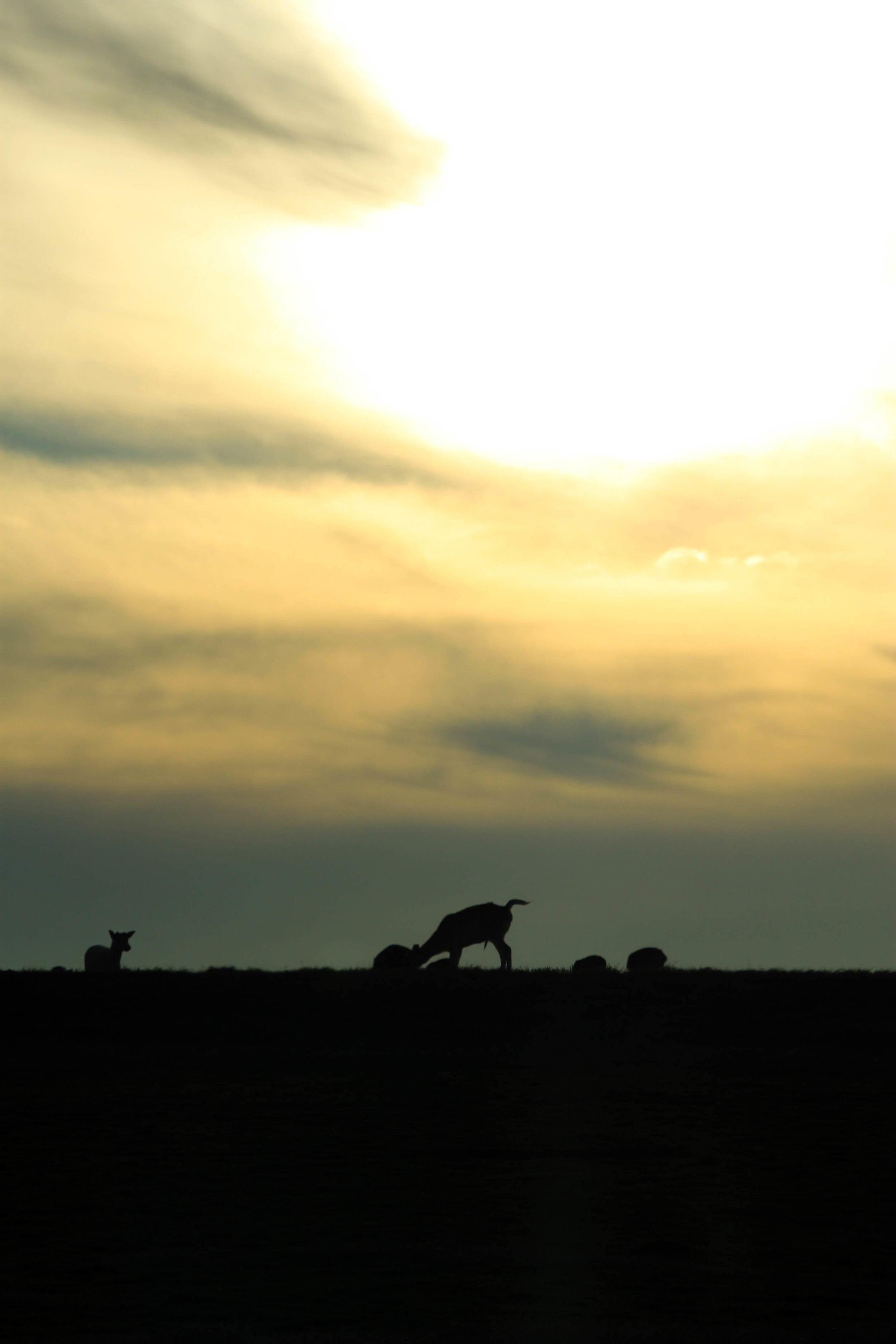This photograph captures a serene, dusky landscape dominated by a vast sky rich in color gradients. About two-thirds of the image is filled with a dramatic sky, transitioning from an intense orangish-yellow with dark grey clouds at the top to a dusky grey or blue near the horizon. This suggests it’s either dawn or dusk, likely the latter given the moodiness of the light. In the foreground, silhouetted against this vibrant backdrop, are two four-footed animals, which could be goats or deer, standing in what appears to be a grassland or plain. The animal on the left, smaller and positioned further back, has its head raised, gazing towards the center of the image. The larger animal in the middle is bent over, seemingly engrossed in feeding on or inspecting a mound on the ground. The silhouettes of these creatures and the ground they stand on are rendered almost entirely in black due to the low light, creating a striking contrast with the brilliant sky above.